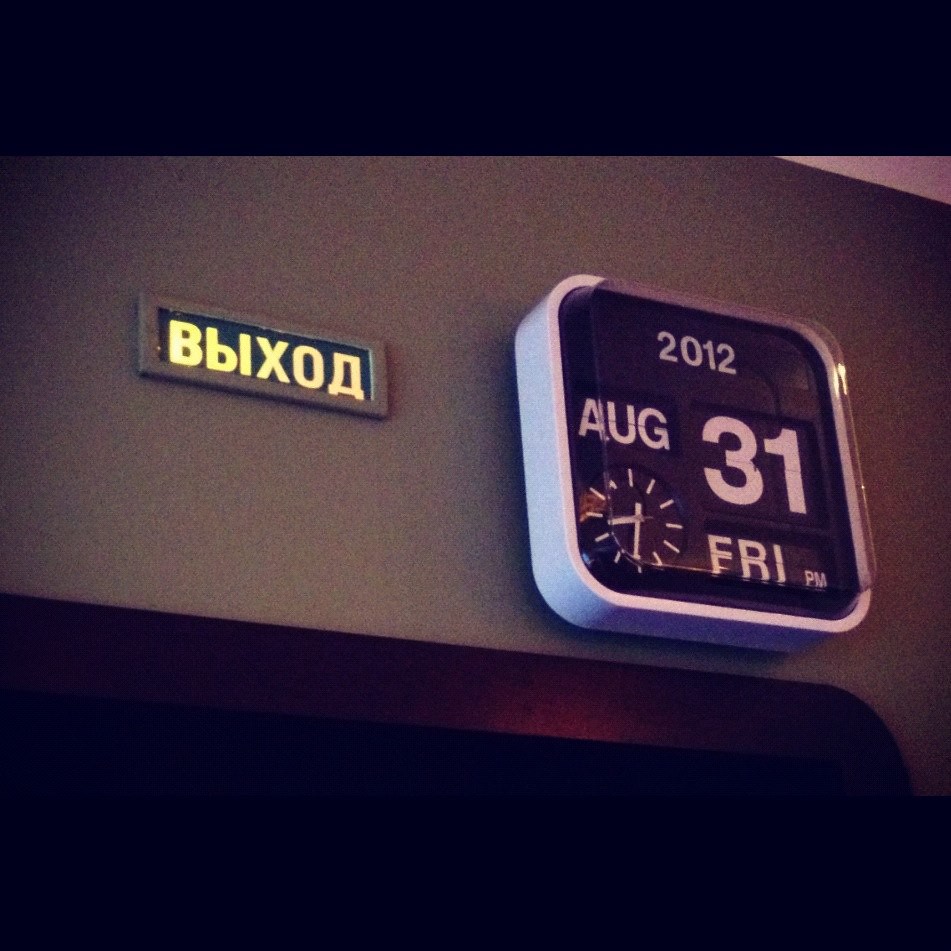The photograph captures a detailed view of a square clock with rounded corners, set against a dark gray background. The clock’s face is black with white text. At the top, the clock displays the year "2012". Below that, "August" and "31" are prominently shown in white, with "31" presented on a flip mechanism indicating the date. The word "Friday" (Fri) and "PM" appear at the bottom, confirming the time as the evening. In the bottom left corner of the clock face, there is a smaller clock without numbers, showing the time as approximately 8:30 PM. To the left of the clock, on a dark brown section that stretches across the background, is a rectangular plaque. This plaque, set in a brown frame with gold letters, reads "BBLXOA". On the far right side of the image, there is a narrow beige triangle, adding an edge to the composition.